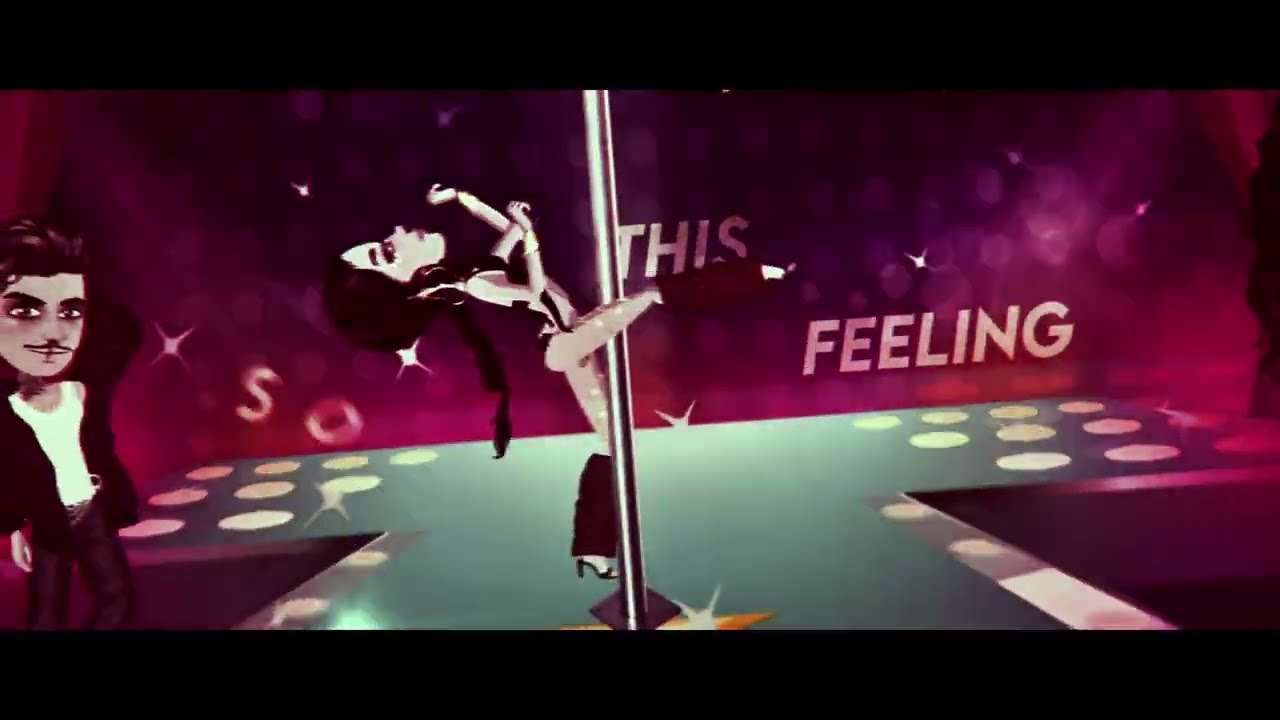In this detailed pop art style illustration, a female pole dancer takes center stage in a visually captivating scene. The dancer, clad in a skimpy black bodysuit resembling a bathing suit, accessorized with high heels and fur-like muffs around her ankles and calves, adopts an intricate pose with one leg wrapped around the pole and her arms raised above her head. Her back is arched dramatically, and her long, braided hair cascades down her back. The stage is bathed in varied lighting effects, with a distinct aqua green striping floor contrasting against a pink-magenta backdrop, which features the partially obscured text "This Feeling" in light pink, italicized lettering emanating from a smoky haze.

On the bottom left of the frame, a man with a modest smile, sporting a thin mustache, a white tank top under a black blazer, dark pants, and curly black hair, is depicted looking towards the camera. He has his hand cupped at the back of his head, adding to the illustrative depth of the image. The entire scene is enhanced with bokeh lighting effects, creating a dreamy and surreal atmosphere that underscores the unique, almost puppet-like animated style of the artwork.